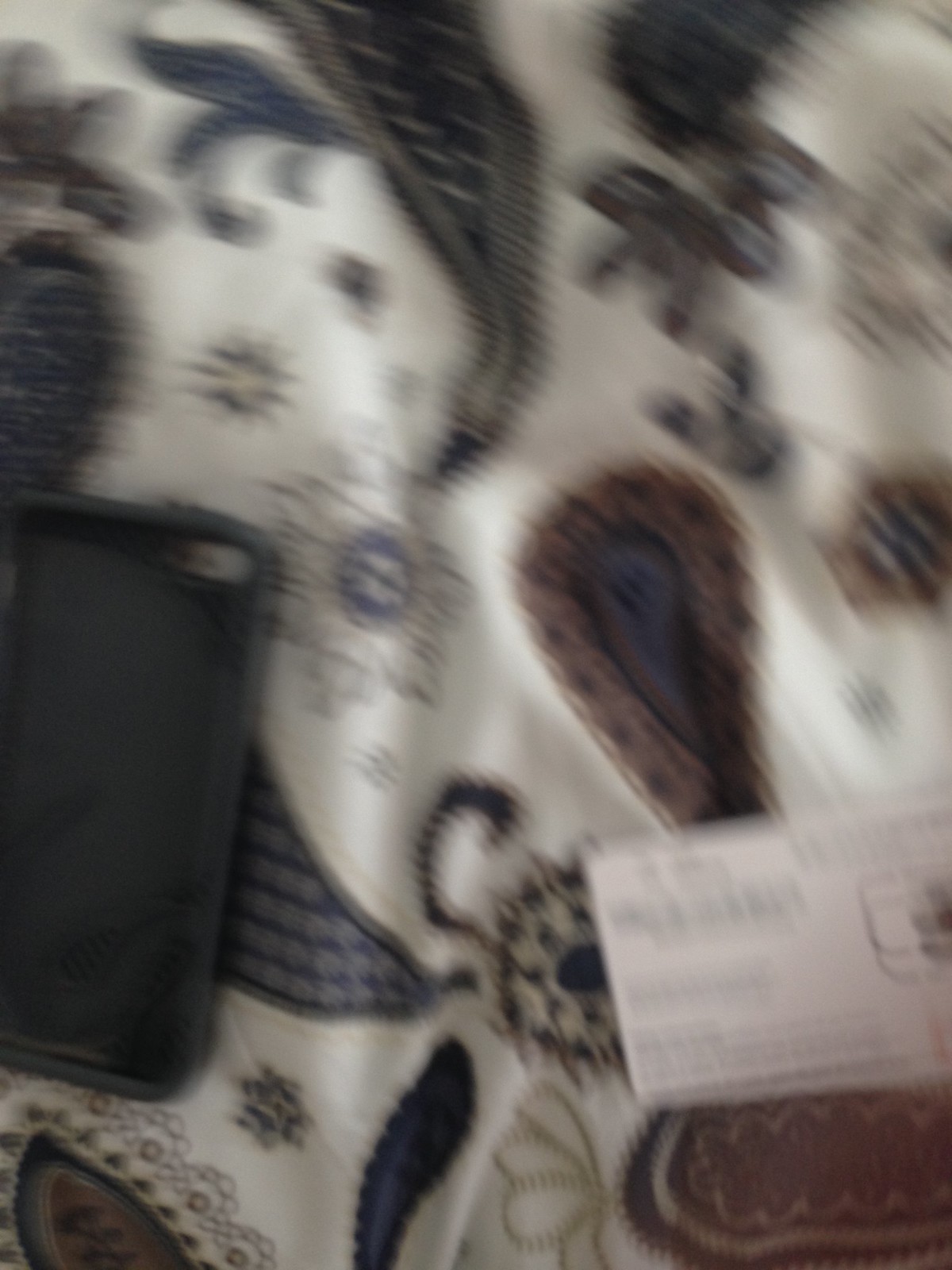This image is an extremely blurry photograph, making it challenging to accurately identify the subjects within it. The photograph appears to depict a table covered with a white cloth featuring various abstract patterns and shapes, including possible blue and brown designs that resemble flowers or floating amoebas. On the left side of the cloth, there is a black rectangle that could be a wallet or a cell phone, but its indistinct nature makes it hard to determine definitively. In the lower right-hand corner, a white piece of paper, potentially a ticket to an event or an envelope with writing and a small square on it, can be seen amidst the blur. Overall, the image's focus issues, possibly caused by a smudge on the lens, leave many details vague and unclear.